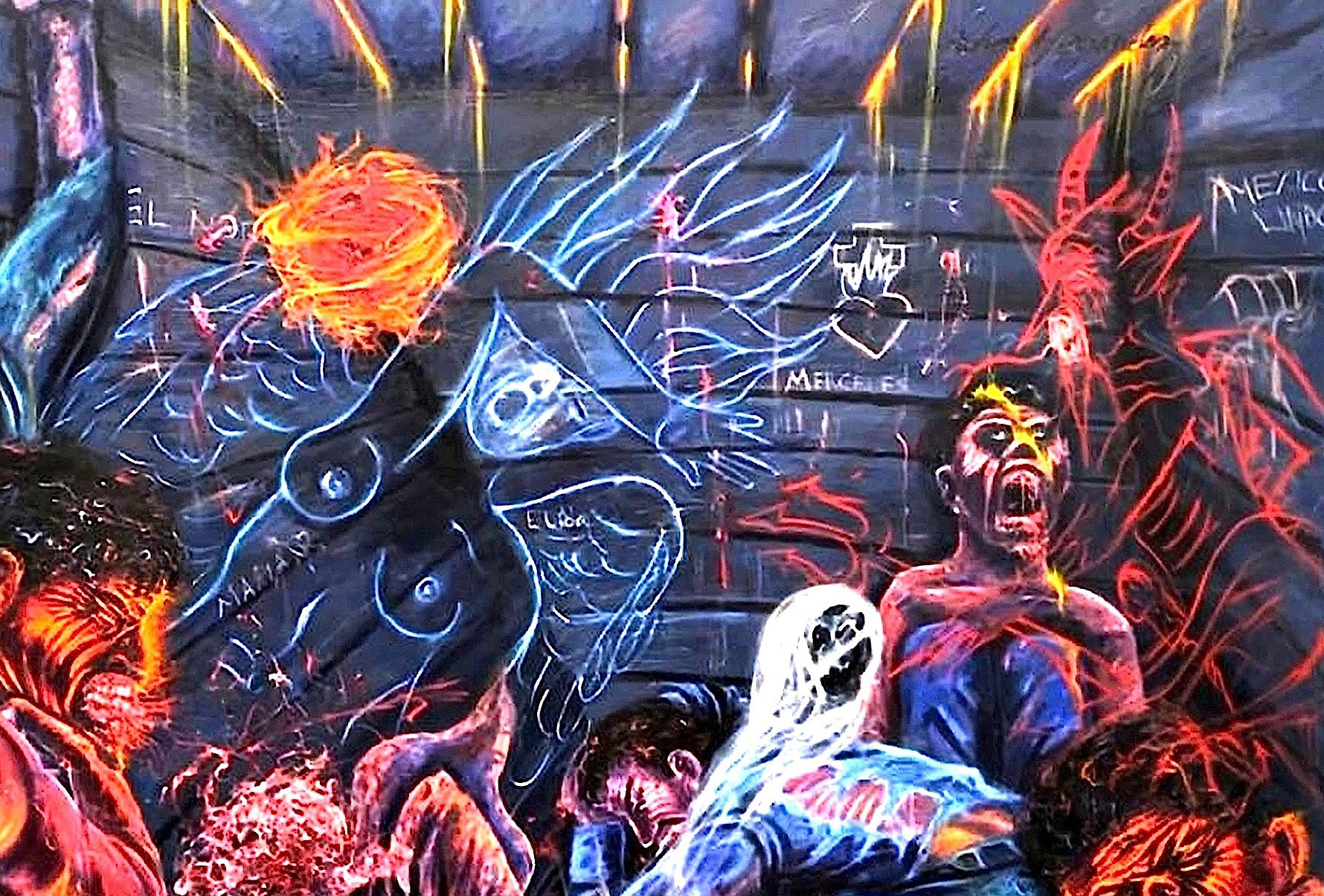The image depicts a sinister and surreal scene possibly representing an artist's depiction of hell. The background is primarily blue, contrasting sharply with the various monstrous and ghostly figures scattered throughout. One particularly eerie figure resembles the iconic "Ghostface" from the Scream franchise, complete with a gaping black mouth and hollow eyes, while another creature, with sharp teeth, has objects hanging from its mouth. Hands protrude ominously from different parts of the image, suggesting a sense of trapped souls and torment.

Set within a structure that resembles a wooden shed made of horizontal planks, there is yellow substance dripping from the ceiling, adding to the unsettling atmosphere. Among these horrors, a prominent figure stands out—a possibly female outline with a triangular head, bare chest, and fiery or hair-like flames emerging from her head, perhaps symbolizing a fallen angel.

On the right side of the image, a devil-like figure colored in red with horns and a tongued pitchfork presides over the scene, adding to the sense of dread. Beneath this demonic overseer, people are depicted in various states of agony, with open mouths screaming in eternal misery. At the center, one tormented soul crouches down, seemingly overwhelmed by pain.

Overall, the image is a detailed, abstract composition filled with creatures, tortured souls, and eerie symbolic elements, featuring an inscription "Emmy" in the top right corner.